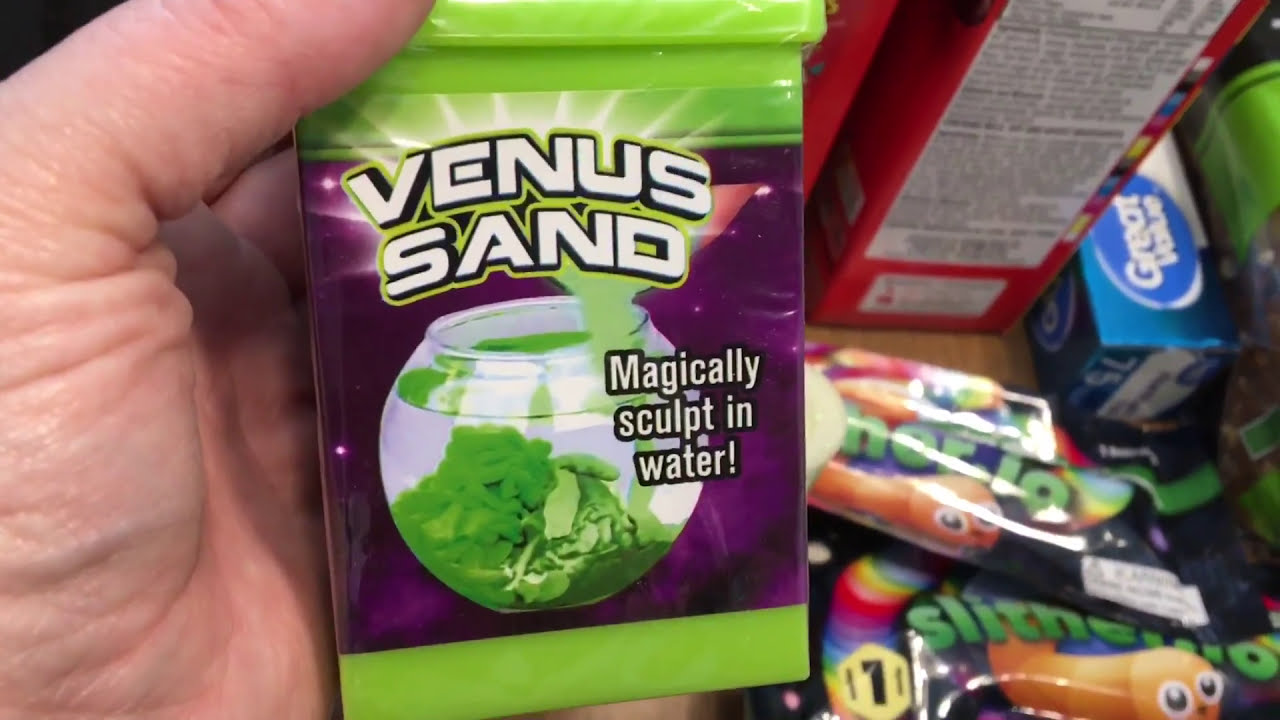In this detailed photograph, the palm of a white man's hand is prominently featured, holding up a lime green rectangular plastic package. The package, labeled “Venus Sand,” has a vibrant purple background with white letters bordered in black and a lime green border framing the text. The label also reads “magically sculpt in water” and features an image of a clear glass fishbowl filled with the green sand. In the background, various other products are partially visible and out of focus, including the Great Value logo on a blue package, which appears to be aluminum foil, along with an assortment of other brightly colored packages, possibly including off-brand gummy worms and other items. The overall scene captures the close-up of the Venus Sand product against a cluttered backdrop of miscellaneous store items.